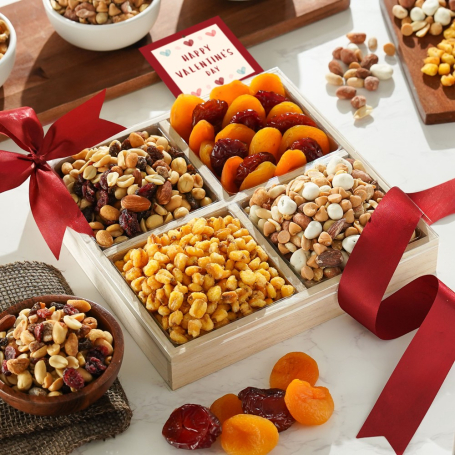The photograph showcases an artistic Valentine's Day arrangement featuring a square wooden box with four separate compartments. Each compartment contains a unique selection: one with mixed nuts, another with dried corn, a third combining nuts and white chocolate, and the fourth filled with dried apricots and prunes. The box is adorned with red ribbons in the upper left and lower right corners, and sits atop a pristine white marble countertop. Complementing the central box, small wooden bowls of dried fruits and nuts are artfully placed around it. At the top of the image, a red card with the message "Happy Valentine's Day" adds a festive touch. The overall presentation is clean, detailed, and designed to highlight the delicious variety of treats, emphasizing the warm hues of orange and brown against the white background.